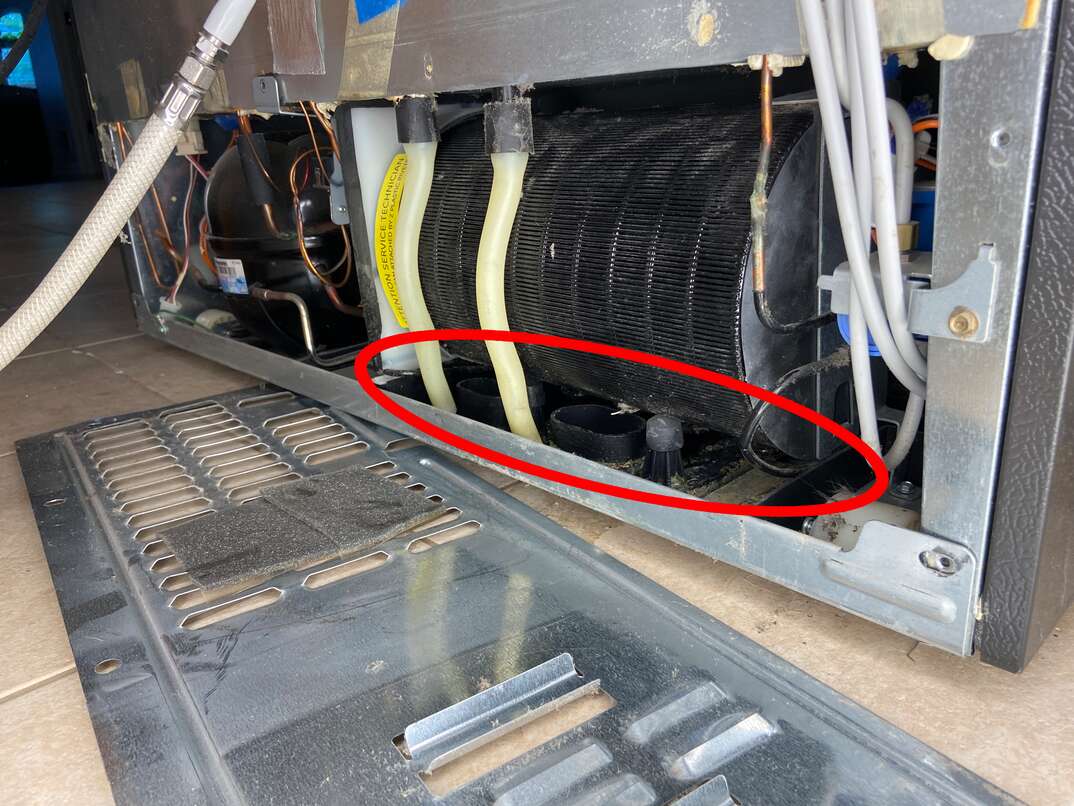The image depicts an indoor scene with a large metal machine, resembling the back of a refrigerator, situated on a beige tiled floor. The back panel of the machine is removed, revealing the inner components. Among these, two black electric motors and several wires and tubes are visible. White wires, appearing more like tubes, emerge from the right side and lead upwards, while two yellow tubes, likely for liquid transport, run in front of one of the tubular-shaped electric motors. Additionally, a white and silver hose is attached to the machinery on the left side. Silver and blue tape is noticeable on the machine. A metal vent door lies on the floor, partially unscrewed, indicating it has been taken off. A prominent red circle, drawn with a magic marker, highlights an area just below one of the black motors, suggesting it needs repair or attention.